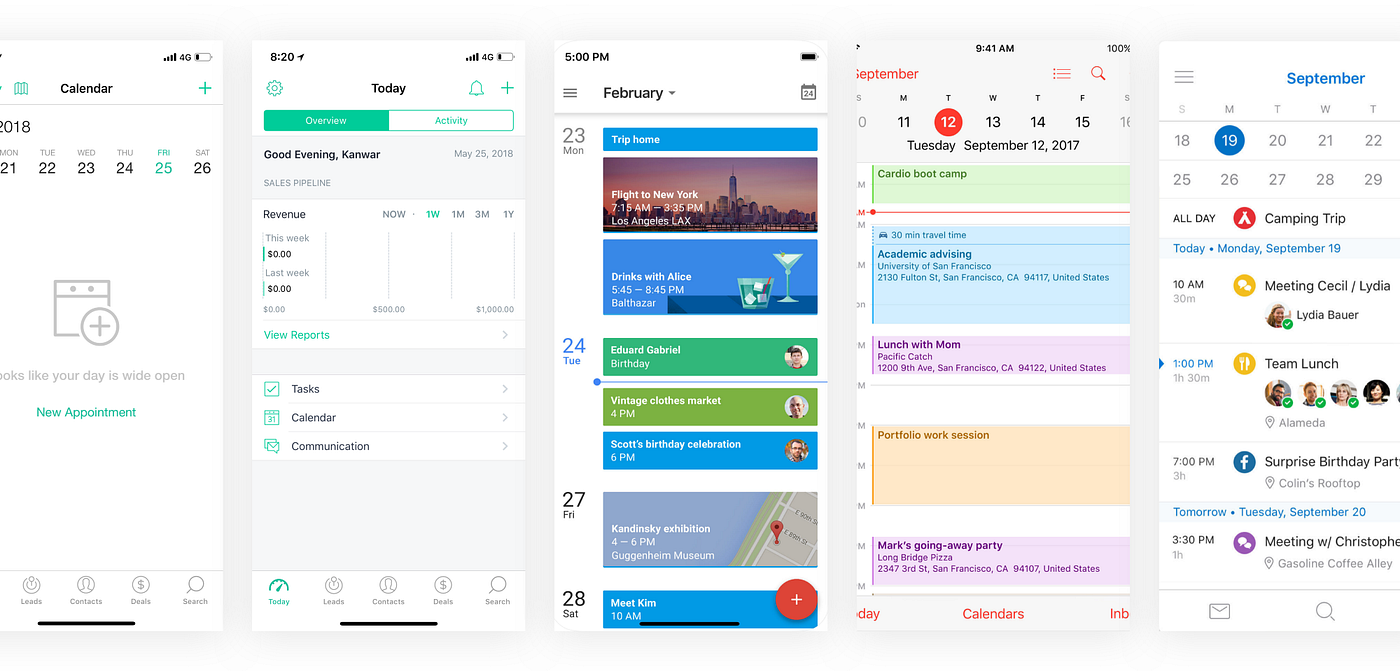The image consists of five screenshots of a phone interface, all related to a calendar application. 

1. The leftmost screenshot displays a calendar interface with the title "Calendar" at the top, showing the year 2018. The date range includes Monday through Saturday, spanning from the 21st to the 26th, with the 25th highlighted. The middle section mentions a new appointment.

2. The second screenshot is labeled "Today" and features sections for "Overview" and "Activity," with "Overview" being highlighted. It greets the user with "Good evening, Canwar." Below this, it shows revenue metrics with both this week and last week listed as zero. The lower part includes tabs for "Tasks," "Calendar," and "Communication."

3. The third screenshot indicates the month of "February." Featured dates include:
   - February 23, Monday: "Trip home, flight to New York from Los Angeles (LAX)" and "Drinks with Alice from 5:45 PM to 8:45 PM at Balthazar."
   - February 24, Tuesday: "Edward Gabriel's Birthday" and "Vintage Clothes Market, Scott's Birthday Celebration."
   - February 25, Friday: "Kandinsky Exhibition."
   - February 28, Saturday: "Meet Kim."

4. The fourth screenshot displays the date "September 12" with various highlighted areas indicating different appointments.

5. The last screenshot shows the month of "September," with the 19th, Monday, highlighted. Appointments listed include:
   - "Camping Trip"
   - "Meeting with Cecil/Lydia"
   - "Team Lunch"
   - "Surprise Birthday Party"
   - "Meeting with Christopher"

This detailed description provides a comprehensive overview of the calendar entries and the interface layout of the phone screenshots.